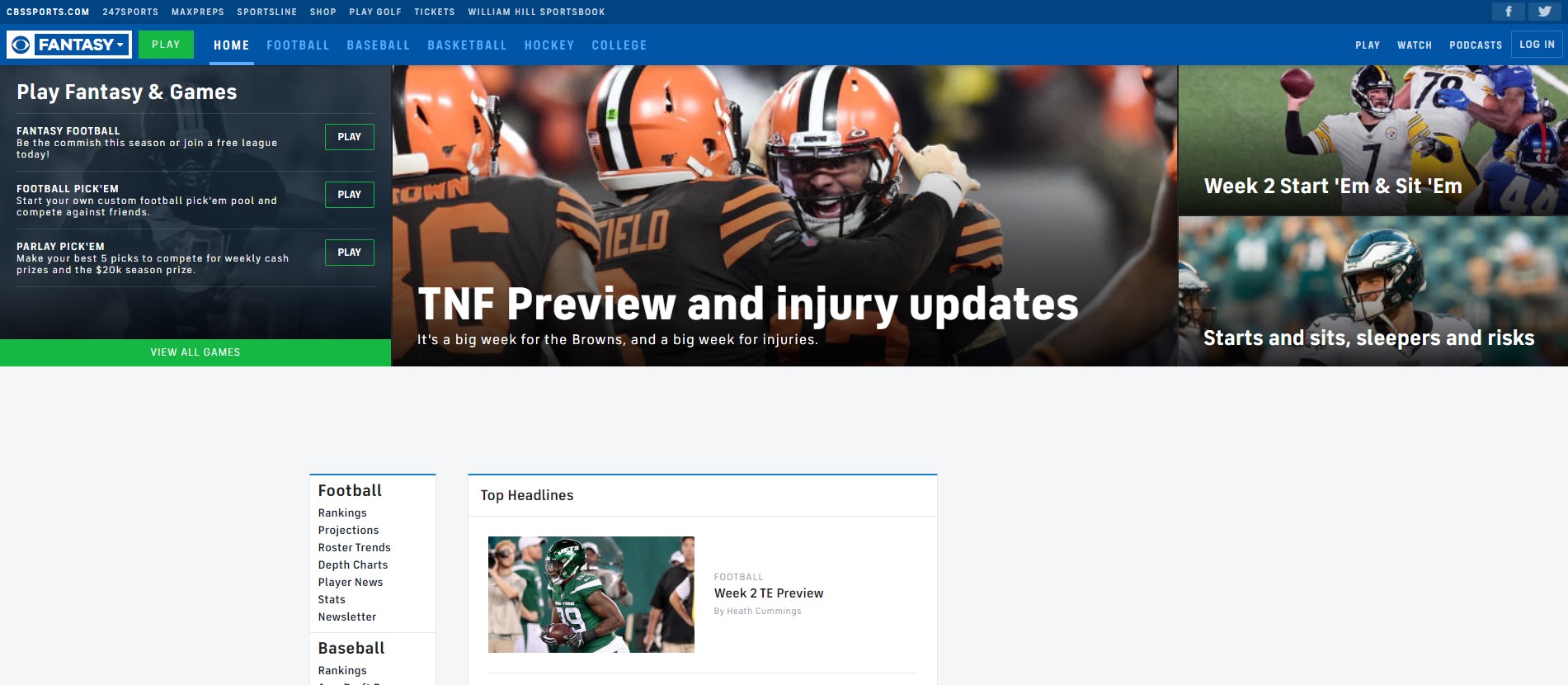The image features a detailed and vibrant layout designed to attract football enthusiasts. The background at the top is a solid blue color, transitioning into a design element on the left—a white and blue rectangle with the word "Fantasy" prominently displayed inside. Below this, in white text, the phrase "Play Fantasy and Games" invites viewers to engage.

On the right side of the image, a group of football players is depicted, all sporting orange, black, and white striped helmets. Notably, one player rests his hand on another's shoulder, while another player's mouth is slightly open, exuding an expression of excitement or intense focus. Below this scene, white text announces "TNF Preview and Injury Updates."

In the upper right corner, an image of a football player wearing a black helmet and a jersey numbered 7 is shown. He holds a football, and beneath him, the text reads "Week 2 Start, Start'em and Sit'em."

A final visual element features another football player in a green and white helmet. The background shows the green stands filled with shadowy figures of spectators, creating a dynamic and energetic ambiance. The caption below states, "Starts and Sits, Sleepers and Risks" in white text, rounding out the comprehensive informational and visually engaging image.